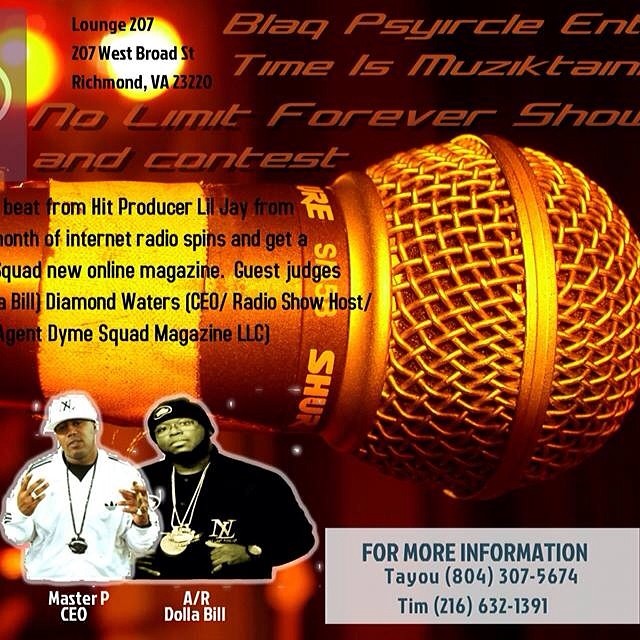This vibrant promotional poster advertises an upcoming rap and DJ contest at Lounge 207, located at 207 West Broad Street, Richmond, Virginia, 23220. Dominated by a striking image of a giant microphone spanning the center, the poster features vivid colors including white, yellow, orange, red, maroon, gold, black, gray, and dark blue, creating an eye-catching backdrop. In the lower left corner, two men pose for the camera: Master P, the CEO, clad in a white Adidas tracksuit with bling, and A.R. Dollar Bill, dressed in a black tracksuit and beanie. The text, though partially obscured, mentions the "No Limit Forever Show and Contest" with a beat from hit producer Lil Jay and promises a month of internet radio spins. It highlights guest judges, including Bill Diamond Waters from Dime Squad Magazine, LLC. For more details, the poster directs readers to contact Tayu at 804-307-35674 or Tim at 216-632-1391. The overall design, style, and details suggest a high-energy event set to take place in a lively club environment.